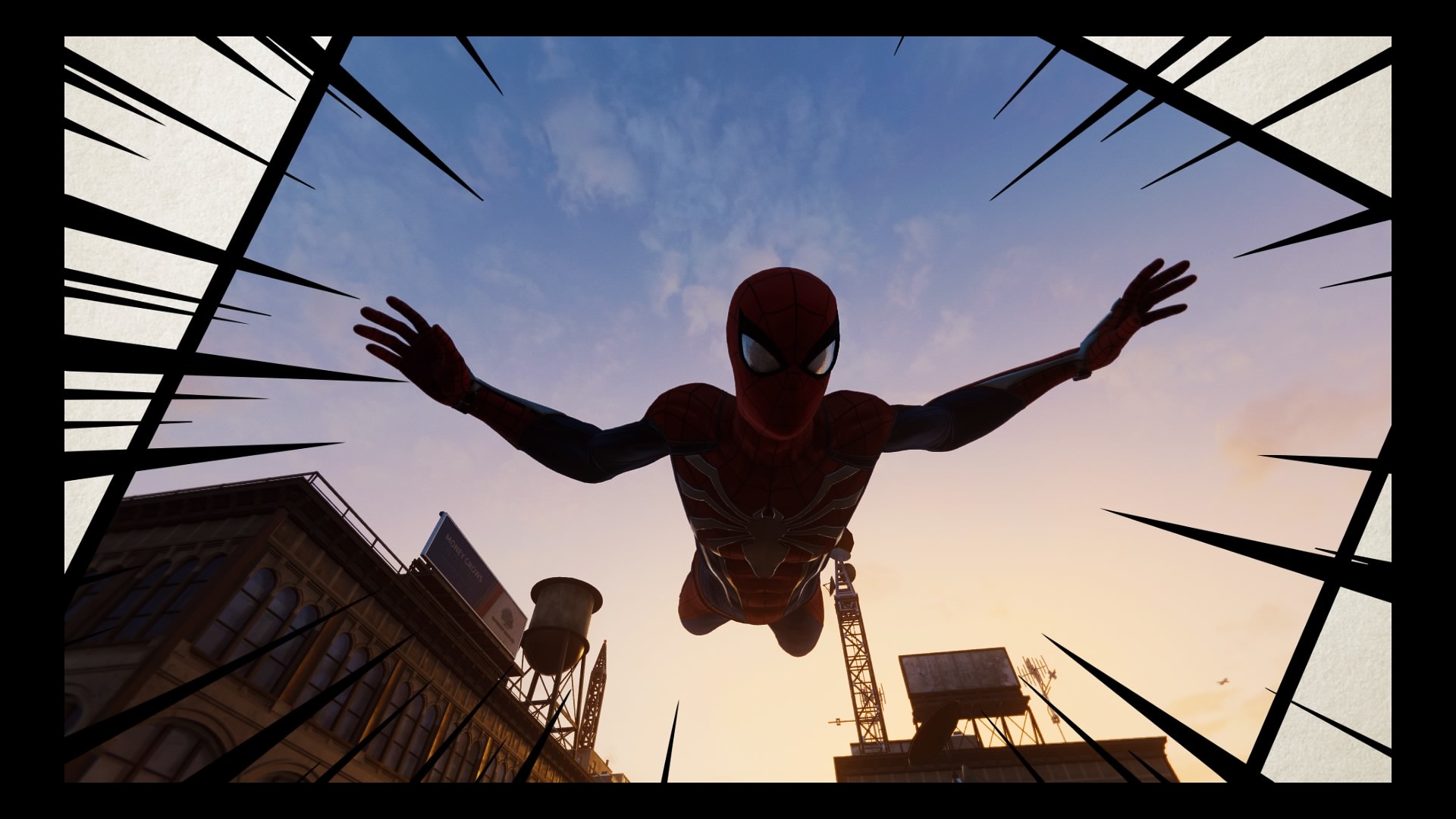In this detailed graphic depiction, Spider-Man leaps dynamically towards the viewer from a building, set against a vibrant and multi-hued sky. His iconic red and blue suit is vividly detailed, featuring an oval red mask with slanted, white, black-bordered eyes, and a noticeable, light-gray spider symbol displayed prominently on his chest. Spider-Man's powerful physique is highlighted with large shoulders tapering into narrower biceps and broad forearms, while his very long fingers are prominently visible. His legs are bent at the knees and point upwards, contributing to the sense of movement. 

The background sky transitions seamlessly from a medium blue with scattered clouds to shades of light purple, pink, blue, and even a hint of light orange towards the right. Two building tops adorned with billboards and a possible water tower or radio tower are visible below, adding depth to the scene.

The entire image is framed within a diamond or square tilted slightly, bordered by a thick black outline. Each corner of this border features black spikes extending inward, emphasizing the dramatic action. Overall, the scene captures Spider-Man in an electrifying moment, hurtling towards the foreground with grace and intensity.